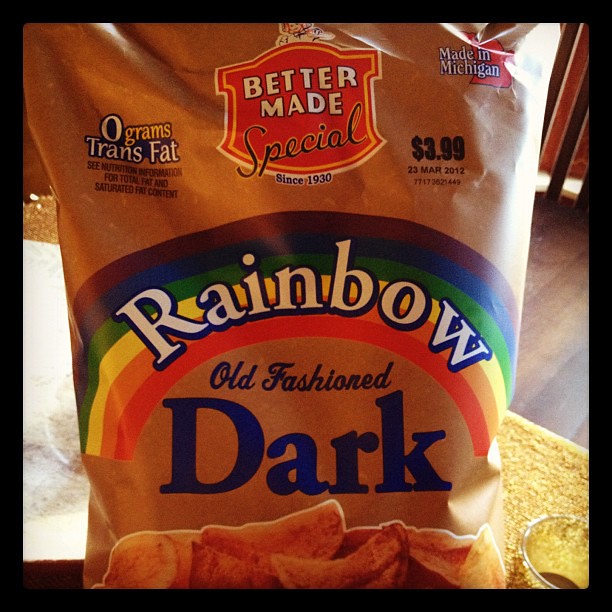The image captures a detailed view of a bag of potato chips. The top right corner prominently displays "Made in Michigan," indicating the product's origin. The top middle section features the brand's emblem, reading "Better Made Special Since 1930," showcasing its long-standing history. On the top left, the packaging highlights a health note: "Zero Grams Trans Fat." The bag is priced at $3.99, with an expiration date of March 23, 2012, clearly marked.

In the middle segment of the bag, a colorful cartoon rainbow is depicted, with the word "Rainbow" in white text imposed over the illustration. Directly below the rainbow, the words "Old Fashioned Dark" are boldly printed, describing the product. The lower part of the bag showcases a representative image of the product, which appears to be dark, possibly kettle-cooked, potato chips. The overall color theme of the bag is a rustic brown, adding to the old-fashioned aesthetic.